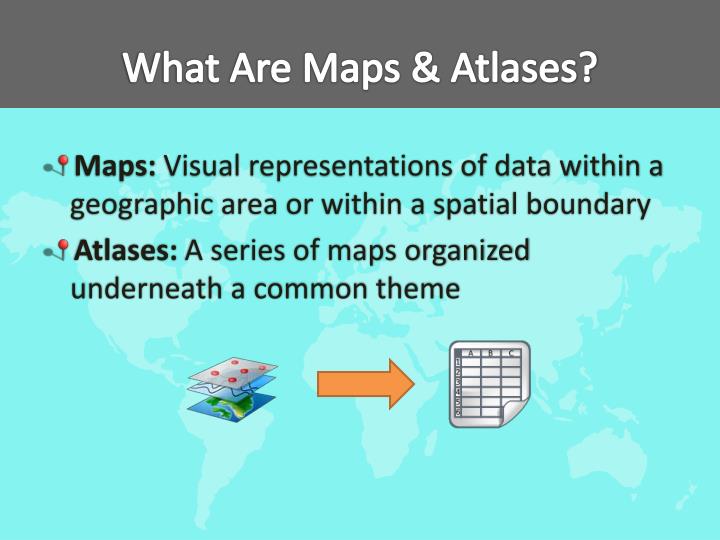The image is a PowerPoint slide with a predominantly blue background and a gray rectangular banner at the top, featuring the white text, "What are maps and atlases?" Below the banner, there’s an image dominated by a teal outline of the world's continents (excluding Antarctica). The text continues in black font with the definition, “Maps: Visual representations of data within a geographic area or within a spatial boundary.” Further down, another text reads, “Atlases: A series of maps organized underneath a common theme.” 

To the left of each definition, there's an icon of a pin with a red head casting a small shadow. At the bottom of the slide, three images are depicted: one showing three overlapping squares (the topmost white with red circles, a lined page underneath, and a map of a small area at the bottom), followed by an orange arrow pointing right, and finally, an illustration of a spreadsheet with rows and columns.